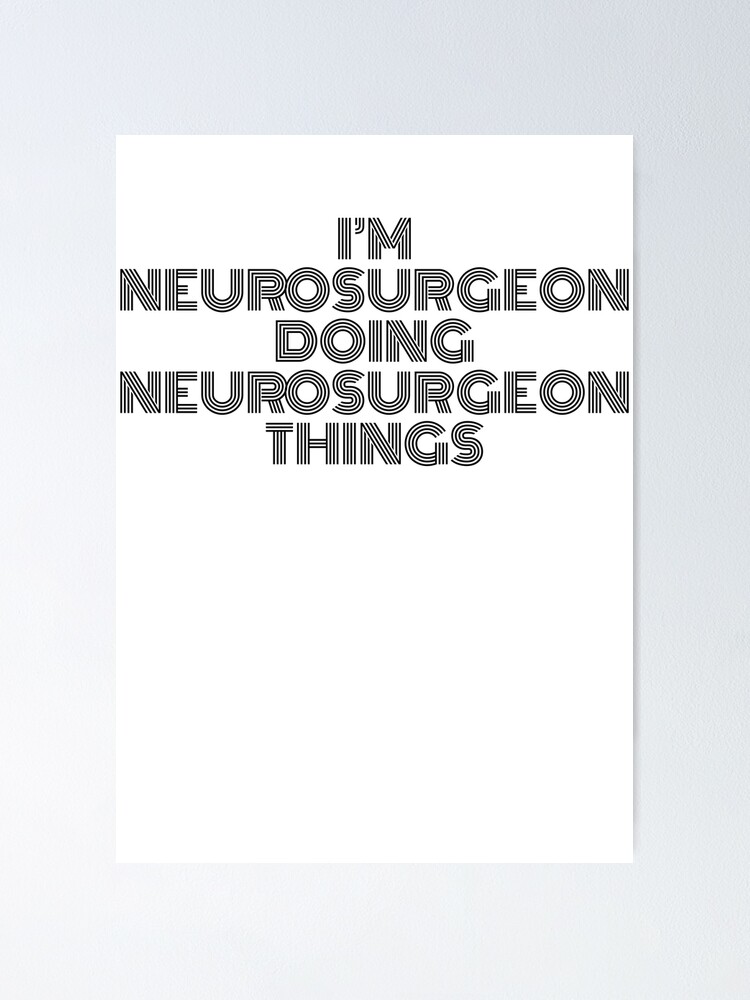The image depicts a piece of wall art featuring a stark, minimalist design. At its center is a rectangular sheet of plain white paper set against a light grayscale background. The focal point of the artwork is the text, which reads, "I'm a neurosurgeon doing neurosurgeon things." The text is uniquely formatted, spanning five lines, with the words "I'm" at the top, "neurosurgeon" on the second and fourth lines, "doing" on the third line, and "things" on the fifth. The font is black, bold, and striped, creating an outline effect. There is no frame around the paper, and the overall composition is simple yet striking, enhancing the stark contrast between the white paper, the bold text, and the pale gray background.